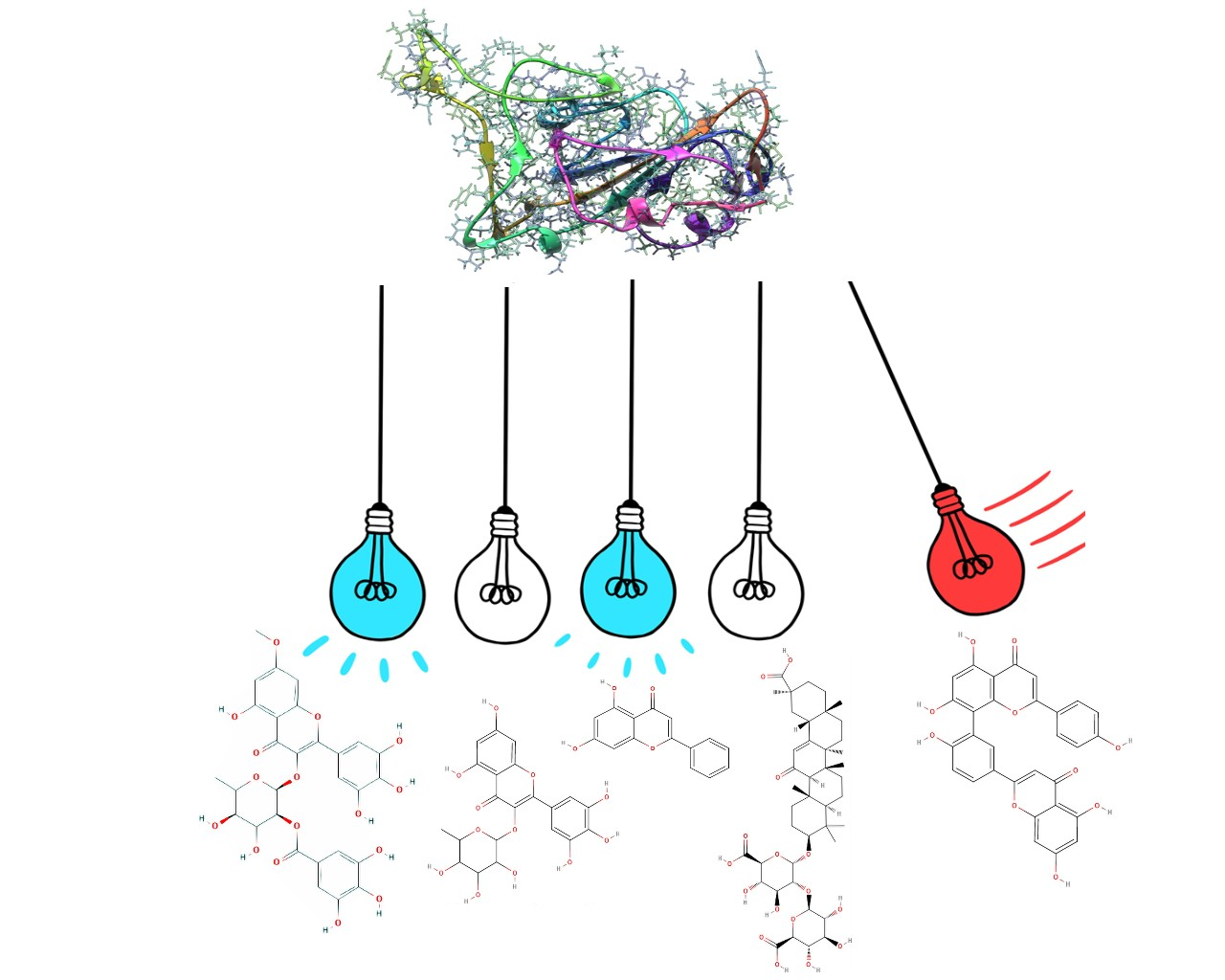The image is a detailed scientific illustration set against a white background. At the top, there is a tangled cluster of multi-colored strands resembling chemical structures or DNA strands, with hues of purple, green, white, and blue. This colorful jumble features overlapping chemical symbols and signs, contributing to a complex, interconnected visual theme.

Beneath this, centrally located, are five light bulbs hanging from partial black wires, which could be imagined as suspended from a ceiling. The light bulbs are arranged in a sequence of blue, white, blue, white, and red. The bulbs resemble classic Edison styles, and their colors and positions suggest a deliberate order. The red light bulb on the right side is distinctively depicted in motion, swinging towards the others like a Newton's cradle, suggesting an impending collision.

At the bottom of the image, there are approximately five cellular diagrams with honeycomb patterns, featuring intricate labels, arrows, and letters that are too small to discern clearly. These diagrams, appearing at an atomic or electrical level, add another layer of scientific complexity to the illustration. This elaborate image combines elements of art and science, showcasing light bulbs, DNA-like strands, and honeycomb diagrams in a visually engaging manner.